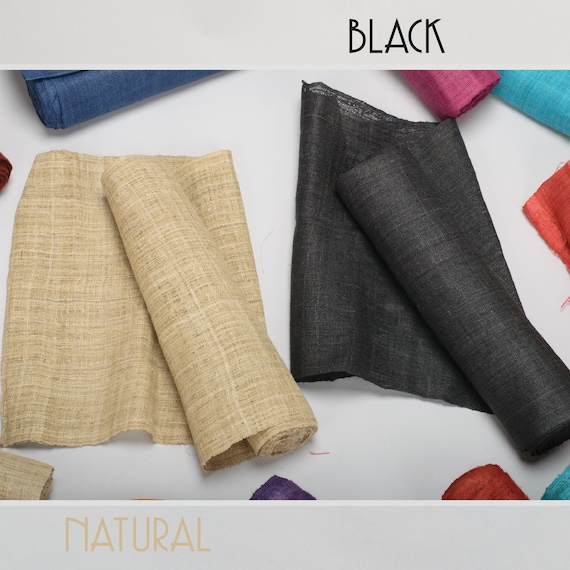The photograph showcases a detailed display of fabric swatches on a white table. The focal point centers on two prominently featured pieces of fabric. At the top, in block letters within a gray banner, the word "BLACK" marks the black fabric beneath it. This fabric is partially stretched out in a square shape with the remaining portion rolled on top. To the left, similarly displayed, is a beige-colored fabric labeled "NATURAL" in matching beige text, also within a gray banner at the bottom. Scattered around the edges of the image are the tips and edges of additional fabric swatches in various colors, including reddish-orange, seafoam green, magenta, deep green, and scarlet. Threads are sporadically strewn across the table, suggesting a dynamic display of textile samples, all of which appear to be crafted from a type of linen or heavy woven fabric.